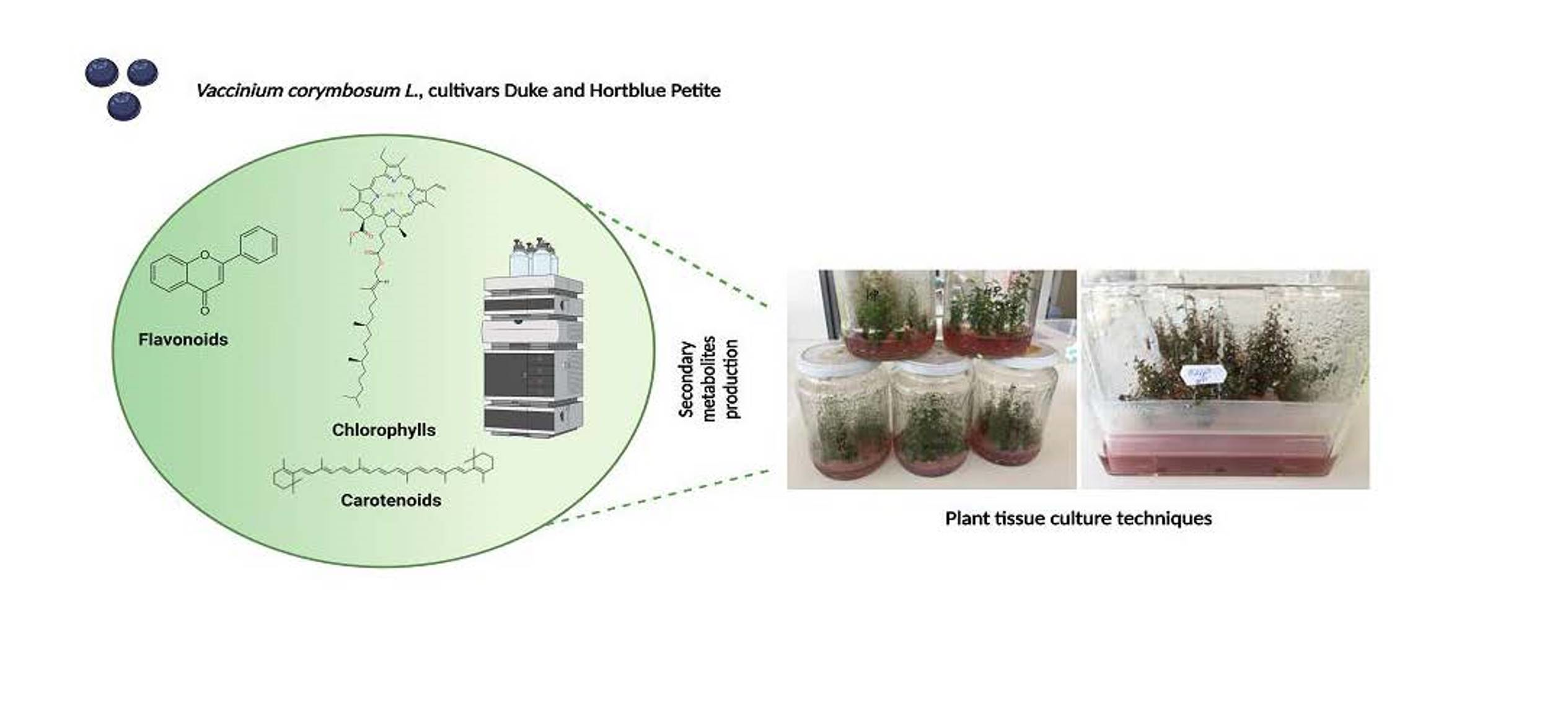This image illustrates plant tissue culture techniques and appears to be taken from a scientific paper or textbook, possibly related to biology. The left side features a detailed graphic design-style diagram with arrows highlighting the production of secondary metabolites, including chlorophylls, carotenoids, and flavonoids, depicted through hexagonal cell structures. The background in this section is blue, and in the top left corner, there are names of blueberry cultivars, such as vicinium, coriandrosum, alkama, duke, and hort blue petite, alongside images resembling blueberries. The right side has two photographs, each demonstrating plant tissue culture methods. The top photo shows a rectangular specimen jar with a red base and a clear leucite lid, containing a plant sample and a white sticker inside. Below it are five containers with red bottoms, arranged with three on the bottom and two stacked on top, all exhibiting significant condensation that obscures the plant life within.